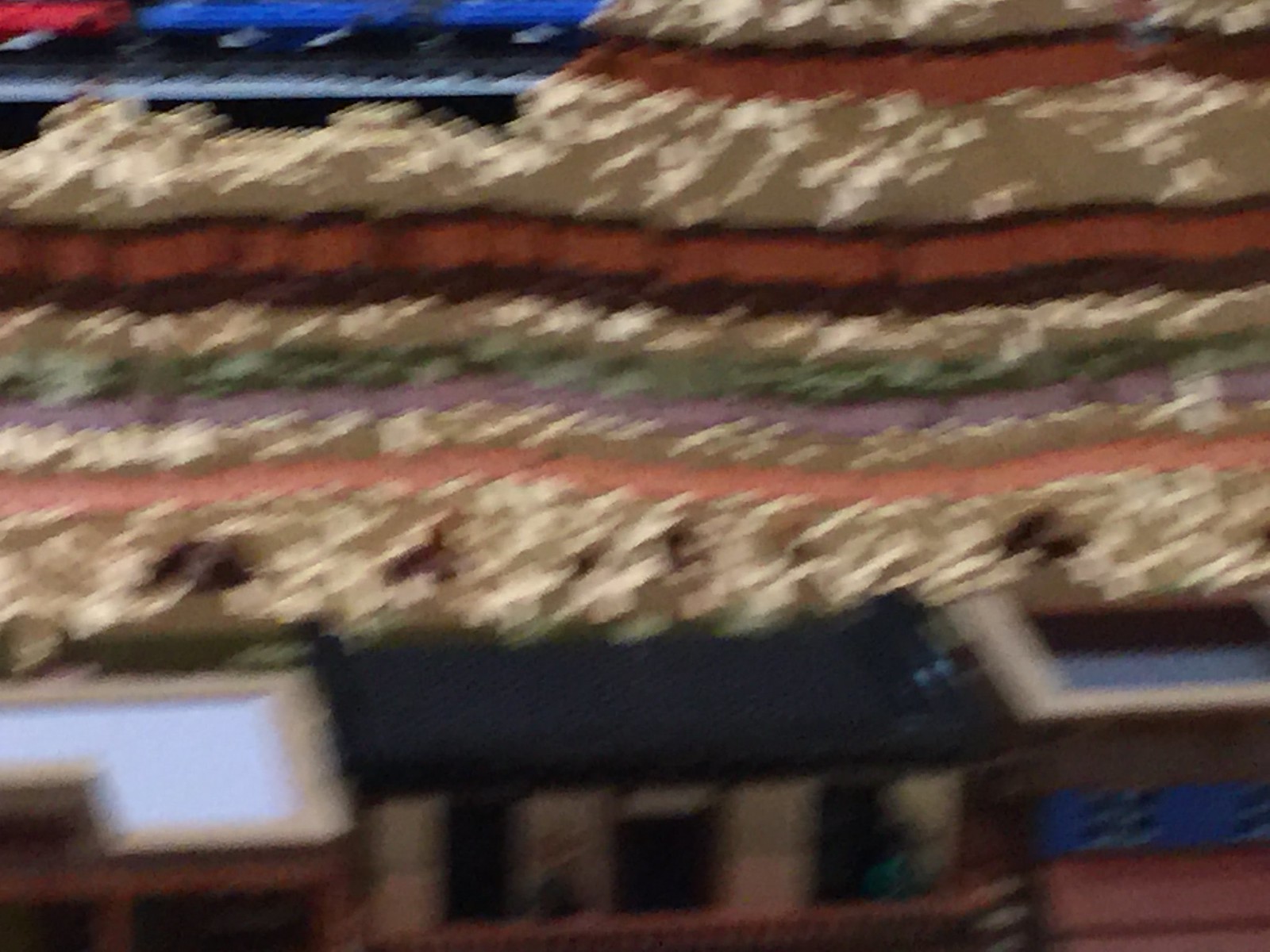This blurry photograph appears to depict a stadium-like setting, though the details are indistinct. On the left-hand side, a structure resembling a soundboard is visible. The center-bottom portion seems to showcase part of a stage, while another possible soundboard is located on the right bottom. The image is layered with various colors—yellow, peach, purple, green, brown, black, and red—possibly representing different sections of the stands. Adding to the lively atmosphere, the colors intermingle in a manner that suggests the presence of people, with what looks like arms raised in unison, reminiscent of a crowd performing "the wave."